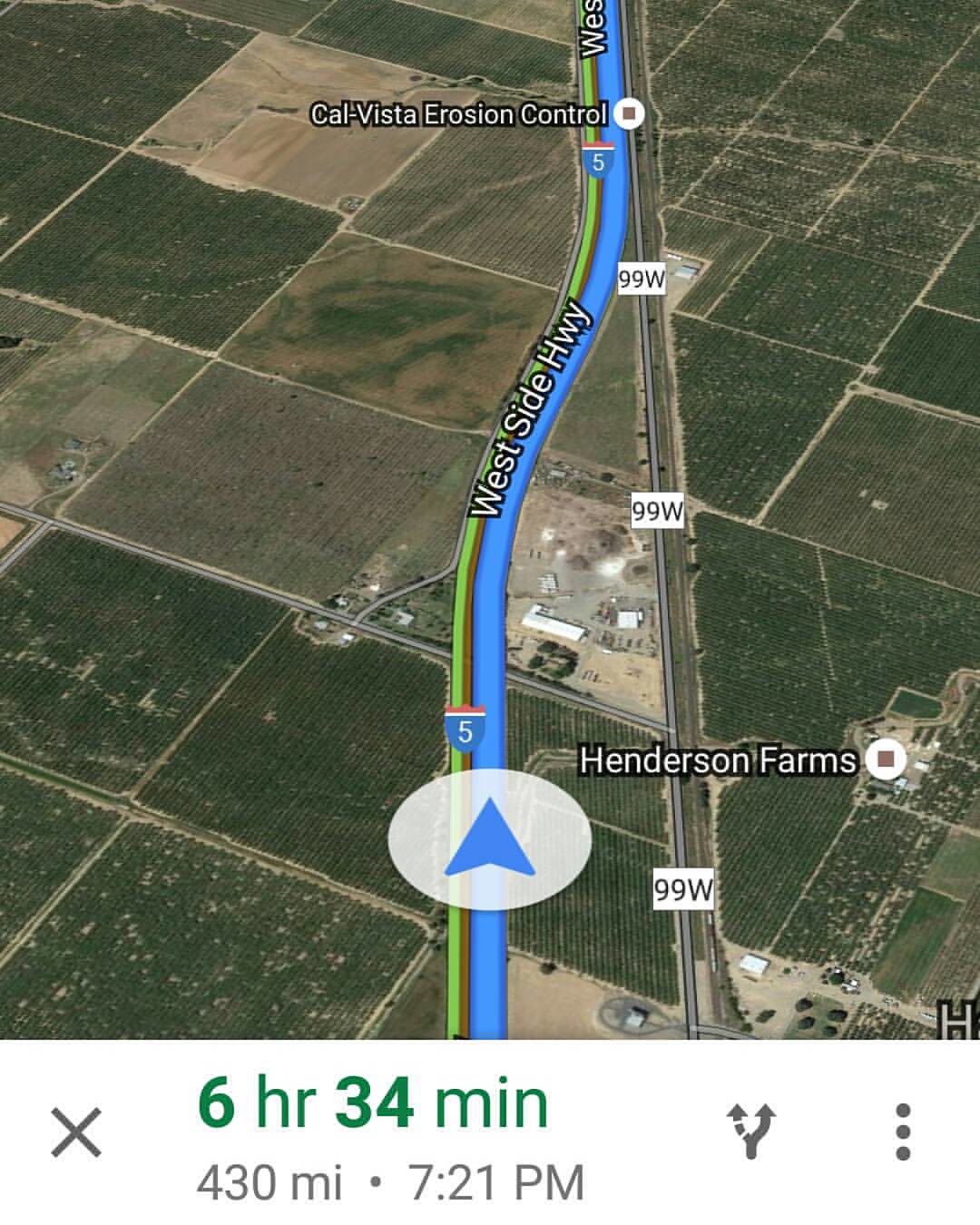The image is a close-up, color-coded screenshot of a satellite view on a navigation app. Predominantly, the image showcases a network of green farm fields organized in square plots. Central to the image is a blue-highlighted route running along a highway labeled "West Side Highway." To the left and right of this highway, various landmarks are annotated in white: "Henderson Farms" lies toward the bottom, and near the top, "Cal Vista Erosion Control" is prominently marked. The route map also includes a green wavy shape adjoining the blue route. Additionally, at the bottom of the screen, the details of the journey are displayed in green font, indicating a duration of 6 hours and 34 minutes, covering a distance of 430 miles, with an expected arrival time of 7:21 p.m.